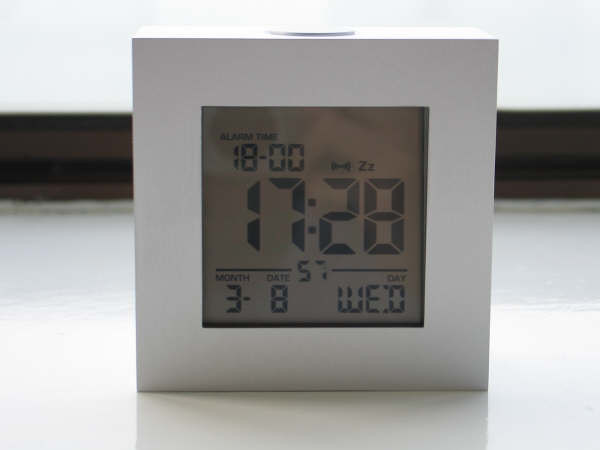This photograph showcases a compact, square digital desk clock with a thick white border and a gray digital display. The clock prominently displays the current time in 24-hour format as 17:28, equivalent to 5:28 PM. The upper left corner of the clock shows an alarm time set for 18:00 (6:00 PM), indicated by a ZZ icon with a bow tie symbol, suggesting the alarm is activated. Below the time, the date is displayed as March 8th (3-8), with "WED" confirming it is a Wednesday. The clock rests on a white reflective surface, with a contrasting black background and a white wall behind it. The design is modern yet quaint, ideal for a desk setup.